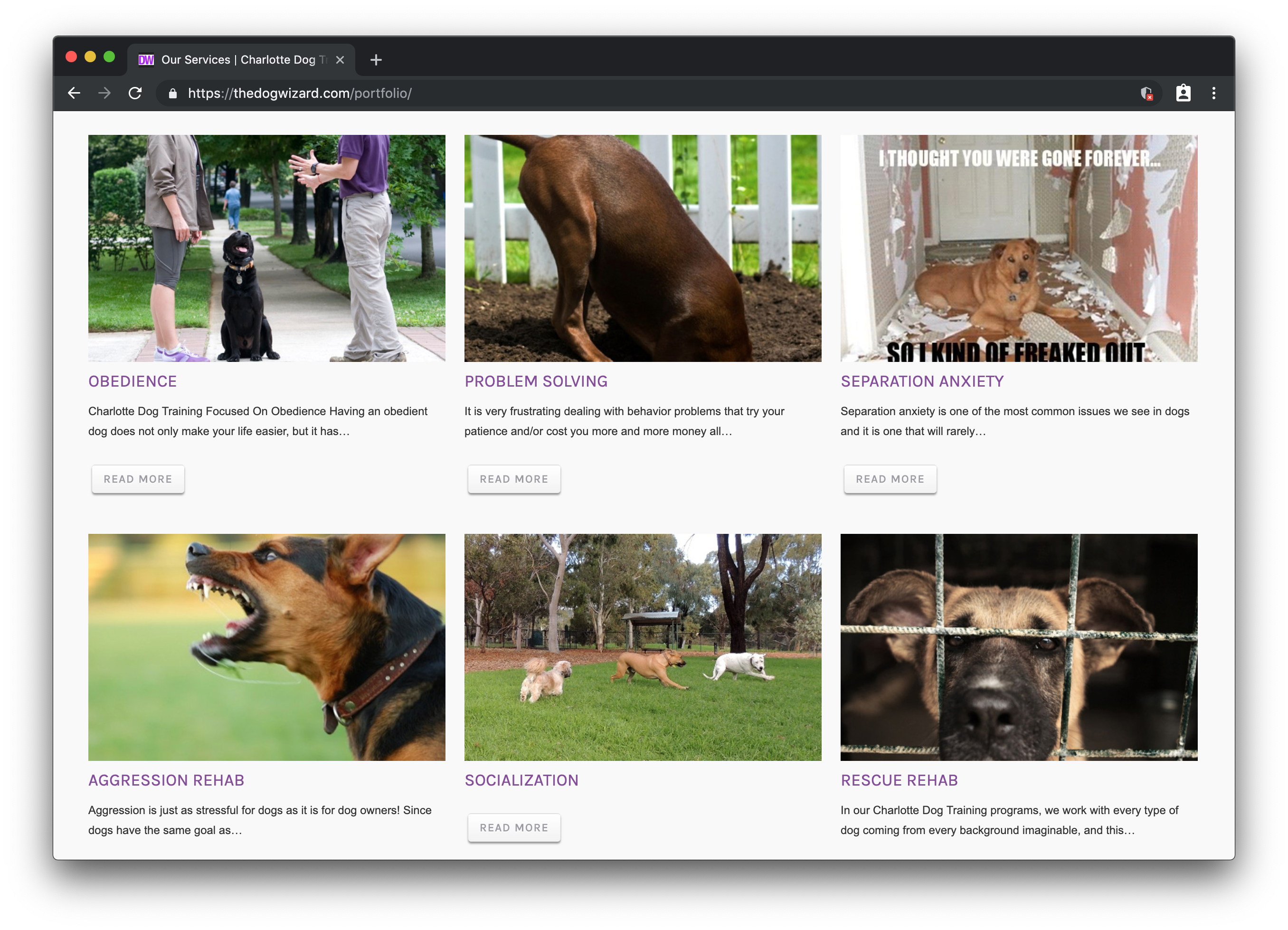Displayed on the screen is a web browser with a sleek black background, featuring three colored circles (red, yellow, and green) at the upper left corner. The browser is focused on a single open tab labeled "Our Service - Charlotte Dog," and the website URL is visible: thedogwizard.com/portfolio. 

The website, with a clean white background, is divided into two rows of content, each containing three images with accompanying text descriptions.

In the first row:
1. **Obedience**: Highlights the importance of having an obedient dog for a more harmonious life. The accompanying text says, "Charlotte Dog Training focuses on obedience. Having an obedient dog does not only make your life easier, but it has..." There's a "Read More" button situated below.
2. **Solving Problems**: Addresses the frustrations and costs associated with dealing with behavior issues. The description reads, "It's very frustrating dealing with behavior problems that irritate patients and/or cost you more and more money. I'll..." Below the text, there's a "Read More" button.
3. **Separation Anxiety**: Features an image of a dog that humorously says, "I thought you were gone forever so I kind of freaked out" while surrounded by torn paper. The text explains, "Separation anxiety is the most common issue we see in dogs and it creates one that will rarely..." with a "Read More" button below.

In the second row:
1. **Aggression Rehab**: Discusses the mutual stress experienced by dogs and their owners due to aggression. The description says, "Aggression is just as stressful for dogs as it is for owners since dogs have the same goal as..." followed by a "Read More" button.
2. **Socialization**: Provides information on the socialization aspect of dog training, with a "Read More" button to explore further.
3. **Rescue Rehab**: Describes their comprehensive approach to working with dogs from diverse backgrounds. The text reads, "In our Charlotte Dog Training program we work with every type of dog coming from every background imaginable and this..." with a "Read More" button below.

Each section invites visitors to learn more by clicking on the respective buttons.